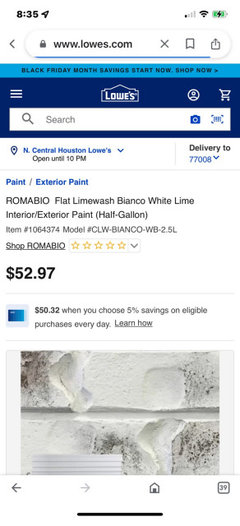A cell phone screenshot of the Lowe's website displays several elements against a white background. In the upper-left corner, black text reads "8:35," with a directional arrow pointing up to the right. The upper-right corner features connectivity bars, a Wi-Fi signal icon, and a battery indicator. Directly beneath, a long white oval contains a left-pointing directional arrow, a small gray padlock followed by "www.lowes.com," an "X" icon, a receipt-like icon, and a square with an upward-pointing arrow inside. 

Below this oval, a blue rectangular banner with a light blue top band and a darker cobalt blue bottom band holds black text stating "Black Friday Month Savings Start Now, Shop Now." Centered beneath this is the white text "Lowe's" along with the Lowe's emblem. 

Next, a long white rectangular search bar features a black magnifying glass icon on the left and the text "Search," with a small blue camera icon on the far right. The line below this indicates "North Central Houston Lowe's, open till 10 PM," and specifies "delivery to 77008."

Continuing downward, it lists "Paint / Exterior Paint" followed by a product description: "Roma Bio Flat LimeWash Blanco White Lime Interior/Exterior Paint (half a gallon)" priced at $52.97. An additional line offers "$50.32 when you choose 5% savings on eligible purchases every day, learn how." 

At the very bottom, an image displays a brick wall painted off-white.